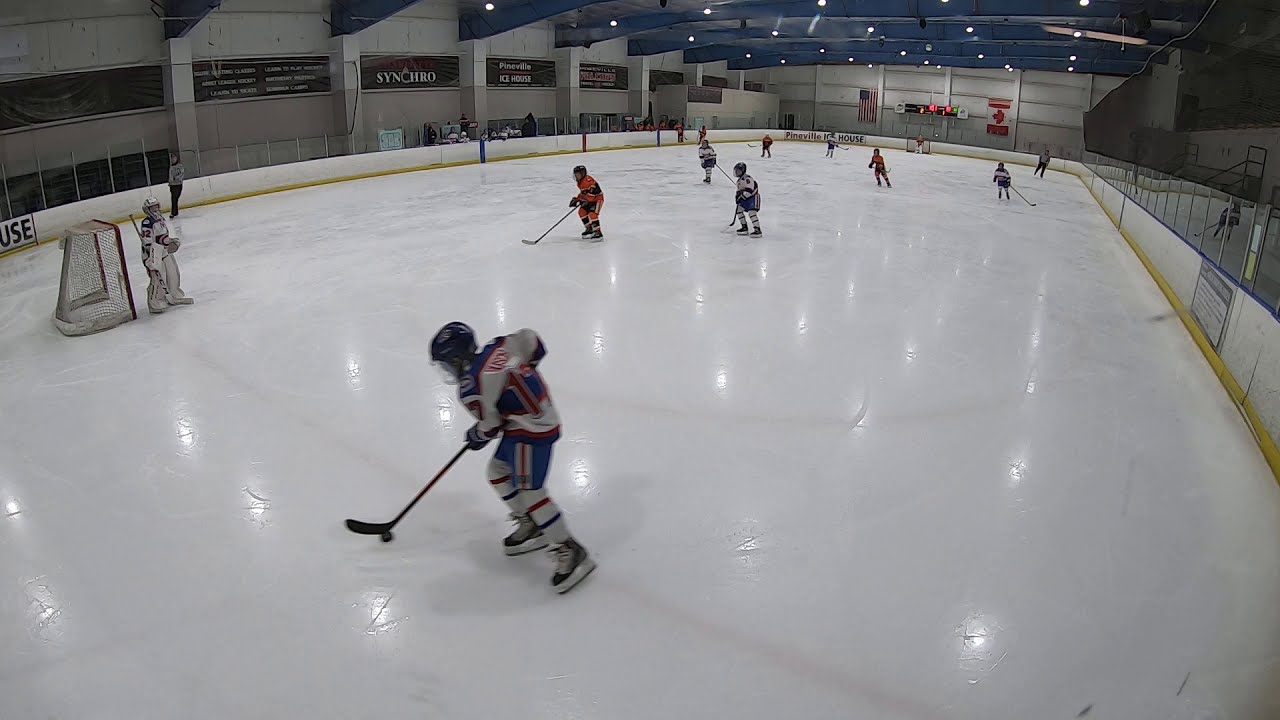This photograph captures a lively moment in an ice hockey stadium, showcasing young kids engaged in a game on a shiny, solid white ice rink. The picture is taken from one end of the rink, providing a wide view from one goal to the other. In the foreground, a young hockey player dressed in a white uniform with blue stripes, red numbers, and text, is seen maneuvering a hockey puck. He is wearing a blue helmet, blue and red bottoms, and black skates, adding to his dynamic presence on the ice.

To the left side of the image, there's a hockey net with a dedicated goalie standing guard and watching the puck intently. Behind him, near the stadium’s boundary, a referee can be seen overseeing the action. The stadium’s walls are adorned with various posters, adding to the vibrant atmosphere. Above, large blue pillars support the ceiling which is equipped with bright lights, their reflections creating a dazzling effect on the ice below. 

On the front wall, prominently displayed, are the flags of the USA and Canada with a scoreboard nestled between them. The scene is lively yet somewhat intimate, with a few spectators visible beyond the rink, highlighting the youthful energy and enthusiasm taking place on the ice.